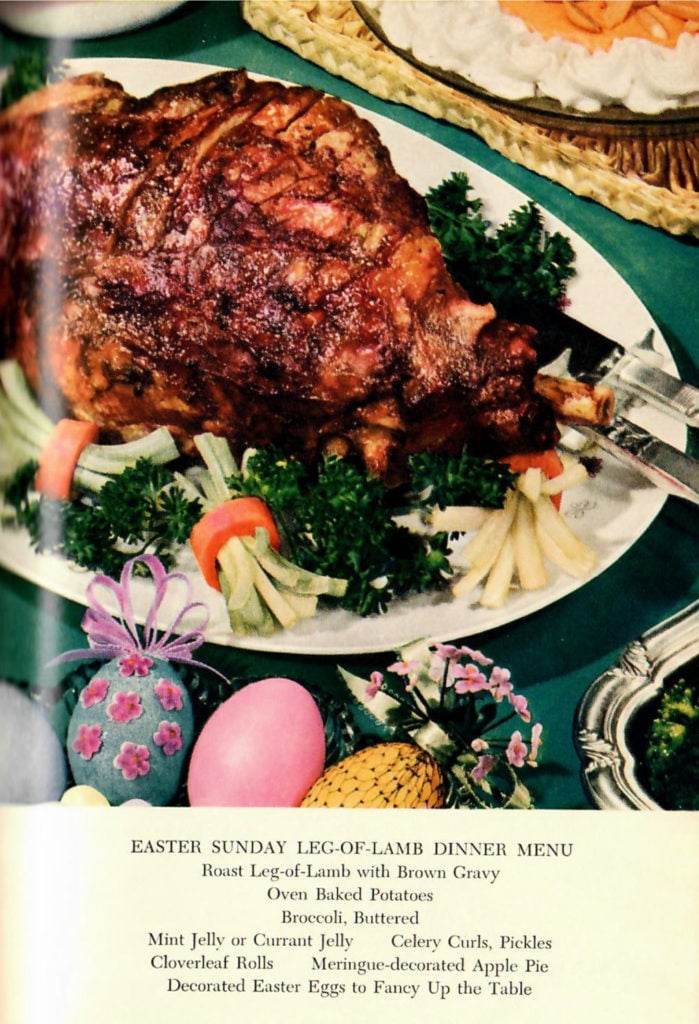The image is a vintage advertisement for an Easter Sunday leg of lamb dinner menu, likely from a cookbook. The centerpiece of the photo is a perfectly roasted leg of lamb, garnished with parsley and thin slivers of celery inserted into hollowed-out carrot rings. Surrounding the leg of lamb are oven-baked potatoes, buttered broccoli, and brown gravy. The table is set with silver cutlery on a dark green tablecloth. The dinner spread also includes mint or currant jelly, celery curls and pickles, cloverleaf rolls, and meringues. 

Notably, there is an assortment of decorated Easter eggs on the table adding a festive touch. The eggs are diverse in color and design: one is periwinkle, another teal with pink flowers and a ribbon, the third is bubblegum pink, and the last is yellow with a black fishnet pattern and pink flowers at the top. A hot plate is located at the top of the image, and a silver tray in the bottom right corner, though its contents remain unclear. An array of accompanying desserts, including a decorated apple pie, are also featured, enhancing the festive and hearty nature of the meal. The image is both detailed and vividly representative of a hearty, festive 80s-style Easter meal setup.